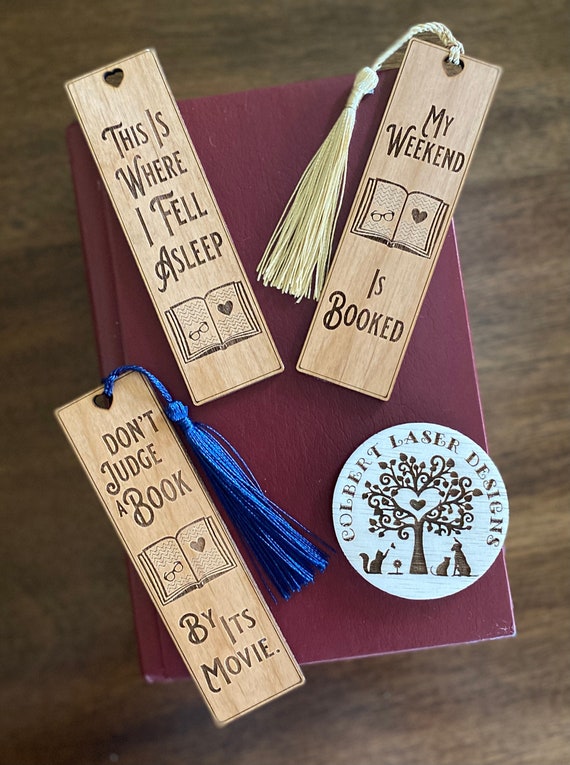The image showcases a product photo from Colbert Laser Designs featuring three intricately laser-engraved wooden bookmarks. Each bookmark is approximately 1.5 inches by 6 inches in size and uniform in material and shape. They are laid out on a maroon-covered book, which lacks a visible title, placed on what appears to be a table or possibly the floor.

The bookmark on the top right has a yellow or cream tassel and displays the inscription "My weekend is booked," accompanied by an engraving of a book with a heart and glasses. The one on the bottom left features a blue tassel and reads "Don't judge a book by its movie," with the same book, heart, and glasses design. The third bookmark, slanted diagonally on the top left, carries the phrase "This is where I fell asleep" but does not include a tassel. 

Each bookmark contains the consistent design of a book with a heart and glasses. Also present is a circular watermark or logo for Colbert Laser Designs, featuring a tree with a cat, dog, and a bird underneath, symbolizing the brand. The logo is in brown and white, reinforcing the natural aesthetic of the wooden bookmarks.